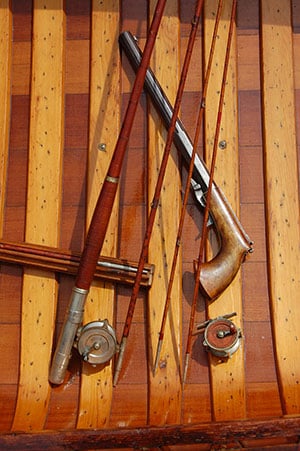The photograph captures a rich, brown wooden boat with alternating dark and light vertical slats, viewed from above. Inside, the boat houses an assortment of timeless, old-fashioned objects. Notably, there are two wooden fishing rods, each equipped with a reel, and a long, single-barrel shotgun with a wooden handle and black barrel, exuding a sense of antiquity. The fishing rods are complemented by two spools, adding to the vintage ambiance. Additionally, there are gold and silver clips visible at the bottom part of the image, with one clip flipped to its side. The scene is bathed in a rich, brown hue with shadows playing across the slats, highlighting the mustard-toned strips and creating a striking contrast. The detailed interplay of wood stains, coupled with the meticulously arranged fishing gear and the shotgun, paints a picture of enduring craftsmanship and rustic elegance.